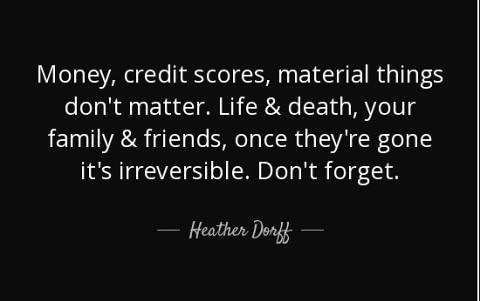The image depicts a small business card-sized rectangle with a solid black background and a thin white border featuring an outer pinstripe. Starting about one-fourth of the way down, there are four rows of white text, properly punctuated, which together form the quote: "Money, credit scores, material things don't matter. Life and death, your family and friends. Once they're gone, it's irreversible. Don't forget." At the bottom, centered along the midline between the fourth row of text and the edge of the card, there is the name "Heather Dorff" in cursive writing, flanked by horizontal dash lines on either side. The overall design is simple yet poignant, emphasizing the message's importance.